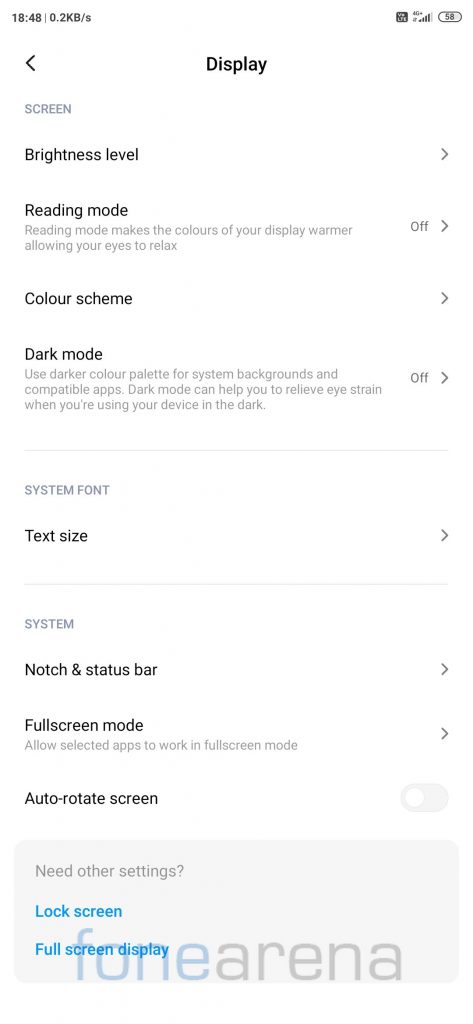Screenshot of a smartphone display settings menu on a completely white background. The interface elements are primarily in black, with select buttons and highlights in blue or gray. The timestamp at the top reads 18:48 in military time. At the top of the list is the "Brightness level," presented with a drop-down menu for adjustment. 

Below it, the "Reading mode" can be toggled on, described as making the display's contours warmer to reduce eye strain. 

Next is the "Color scheme" option, which can be expanded for more settings. The "Dark mode" option is also available, which applies a darker color palette for system backgrounds and compatible apps to alleviate eye strain in low-light conditions; this feature can be toggled on or off and may activate automatically.

Following this, the settings include "System font," "Text size," "System notch," and "Status bar." The "Full screen mode" allows selected apps to utilize the entire screen space. "Auto-rotate screen" and other customizable settings follow.

At the bottom, there are options for "Lock screen" and "Create a full screen display," both highlighted in blue on a gray background. This interface appears to be from a device reviewed on Phone Arena.